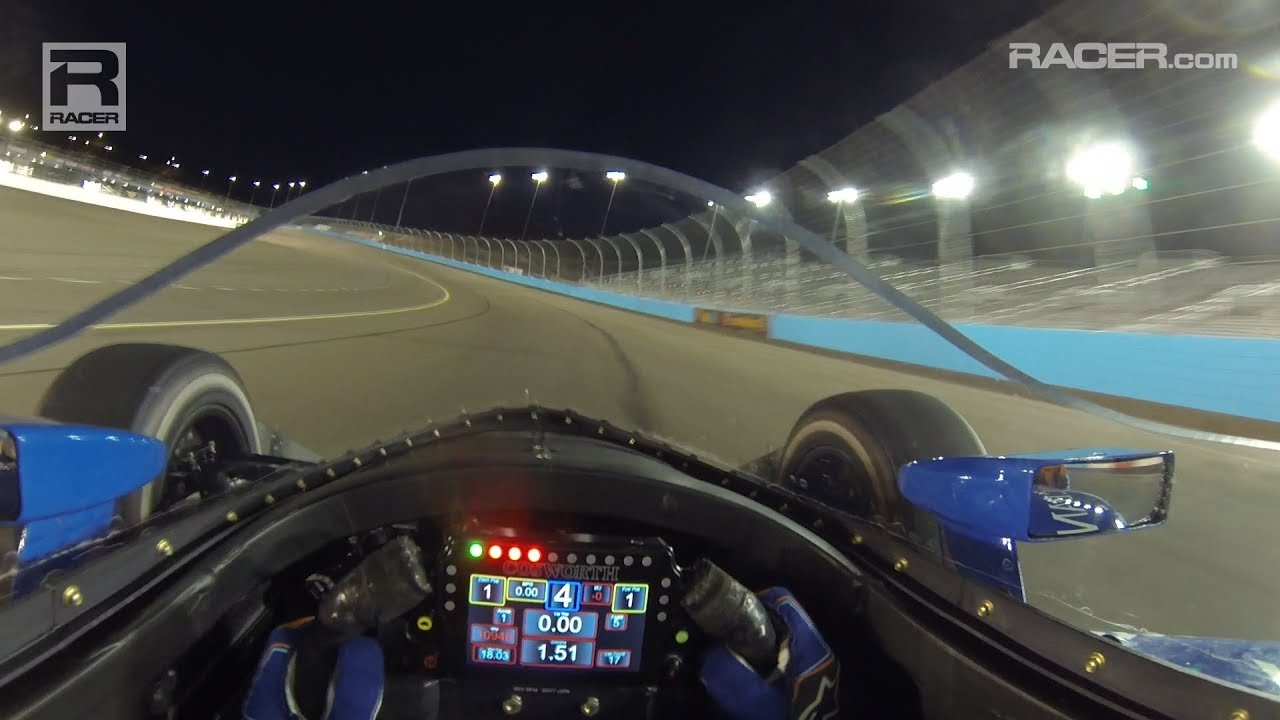The image appears to depict the interior view of a race car, captured either from a photograph or a highly realistic video game. The perspective is from the driver's seat, revealing a dark nighttime setting. The top of the image features a gray text logo on the right side that reads "racer.com" in large letters, with "dot com" in smaller letters. On the left corner, there's an emblem consisting of a black "R" inside a gray rectangle, accompanied by the word "Racer" below in black letters. 

In the foreground, there are two gloved hands gripping a black race car steering wheel. The gloves are dark blue and black. Centrally located on the dashboard is a digital screen displaying various pieces of information, including numbers like "4", "0.00", and "1.51," alongside red and green lights, white numbers, and blue squares. 

To either side of the steering wheel, blue rearview mirrors are visible, alongside the pointy shape of the race car's nose and large black tires. Beyond the car, a dark gray racetrack stretches ahead, appearing slightly blurry. On the right side, a light blue barrier wall topped with wire runs along the track. The stands and additional lights lining the track are also faintly visible, although the stands appear empty. The top left and middle portions of the image reveal a black night sky, enhancing the sense of speed and intensity within the race car's cockpit.